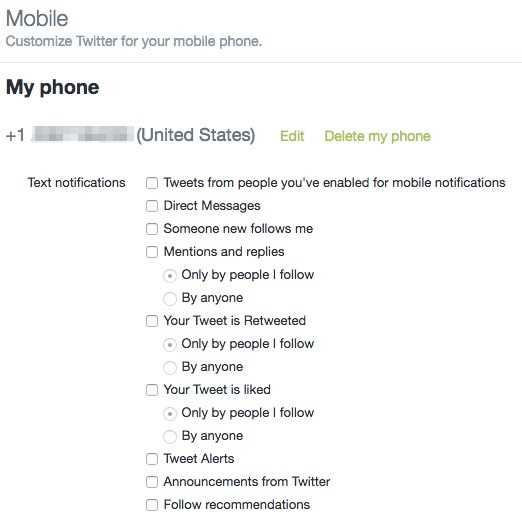The image is a detailed screenshot of a mobile interface for configuring Twitter notifications on a smartphone. 

In the upper left corner, the text "Mobile" is clearly displayed. Below it, there is a label that reads "Customer Twitter for your mobile phone." A thin light gray line runs horizontally beneath the text, separating it from the section below.

Under this line, there's a heading in bold black text that reads "My Phone." Directly beneath it, a redacted phone number is shown with a format similar to "+1 [redacted]," followed by the label "United States." Adjacent to the phone number, there is an "Edit" button and a "Delete my phone" button, both of which allow users to modify or remove their phone details.

Further down, the section titled "Text Notifications" is also in black text and bold formatting. In this section, there are nine primary notification options, each accompanied by a checkbox for user selection and a descriptive label. The options are as follows:

1. Tweets from people you've enabled for mobile notifications.
2. Direct messages.
3. Someone new follows you.
4. Mentions and replies, with subcategories including:
   - Only by people you follow.
   - By anyone.
5. Your tweet is retweeted, with similar subcategories as mentions and replies:
   - Only by people you follow.
   - By anyone.
6. Your tweet is liked.

Each option allows users to customize the types of notifications they wish to receive on their mobile device, enhancing their Twitter user experience. The design is intuitive, with clear text and user-friendly buttons for easy navigation and configuration.